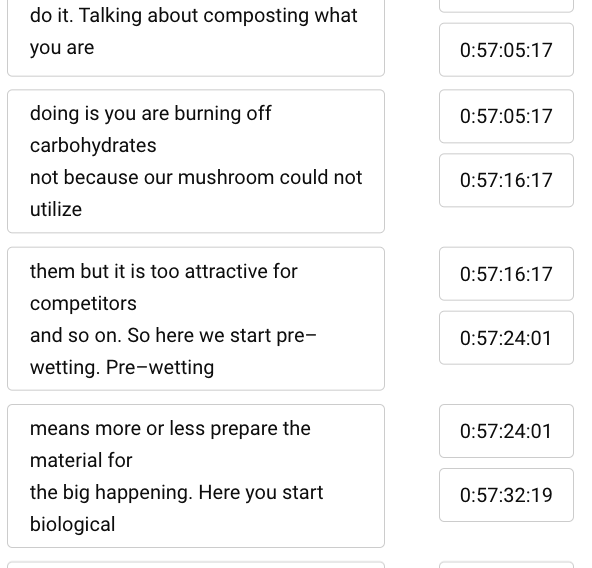This image features a structured white canvas divided into two distinct sections. On the left side, there are four text boxes arranged vertically, whereas on the right side, there are seven similarly arranged boxes.

Starting from the top, the first box on the left side is partially cut off, displaying the text: "Knew it, talking about composting what you are. Talking is you are burning off carbohydrates, not because our mushroom could not utilize them but it is too attractive for competitors and so on. So here we start pre-wetting. Pre-wetting means more or less preparing the material for the big happening. Here you start biological."

On the right side, the seven boxes contain numeric time-stamped data, each punctuated with semicolons instead of colons. They read as follows from top to bottom:
1. Time: 0;57;05;17
2. 0;57;05;17
3. 0;57;16;17
4. 0;57;16;17
5. 0;57;24;01
6. 0;57;24;01
7. 0;57;32;19

This detailed structure suggests a juxtaposition of explanatory text regarding a composting process on the left, and precise time-based data points on the right.